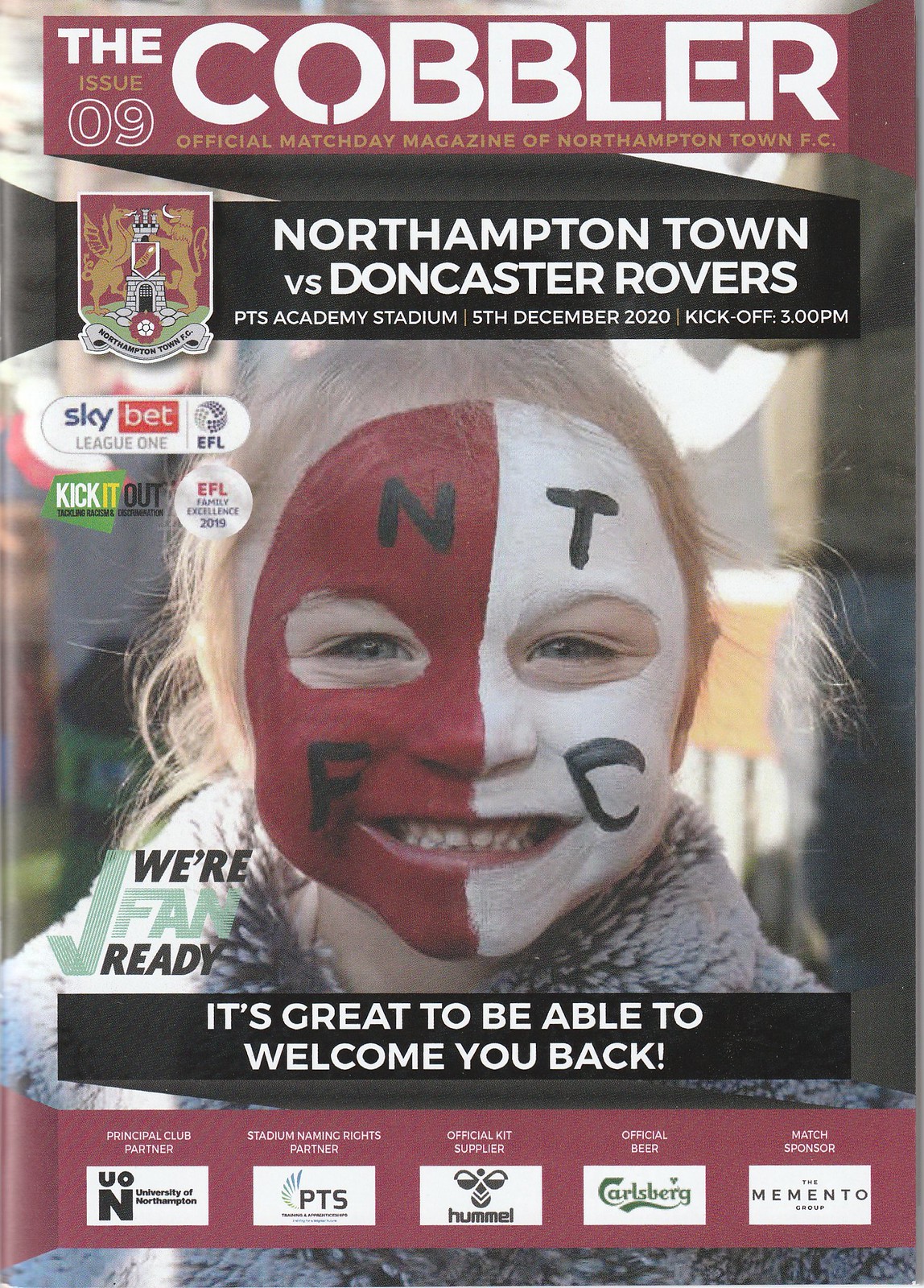The cover of The Cobbler, Issue 09, the official matchday magazine of Northampton Town FC, features an eye-catching design with a prominent maroon stripe at the top. In large, bold white text, the title "The Cobbler" stands out with "Issue 09" and "Official Matchday Magazine of Northampton Town FC" just below it in gold letters. Beneath this, a black banner announces the upcoming fixture: "Northampton Town vs. Doncaster Rovers, PTS Academy Stadium, 5th December 2020, kick-off 3pm."

Central to the cover is a vibrant photograph of a smiling young girl with blonde hair and blue eyes, wearing a fur coat. Her face is strikingly painted—half red and half white—with black letters: "N" on her red forehead, "F" on her red cheek, "T" on her white forehead, and "C" on her white cheek, spelling out "NTFC" for Northampton Town Football Club. The slogan, "We are fan ready, it’s great to be able to welcome you back," adds a warm and inviting touch. The cover is adorned with various sponsor logos at the bottom, such as Sky Bet, EFL, and Kick It Out, completing the detailed and enthusiastic presentation of the magazine.